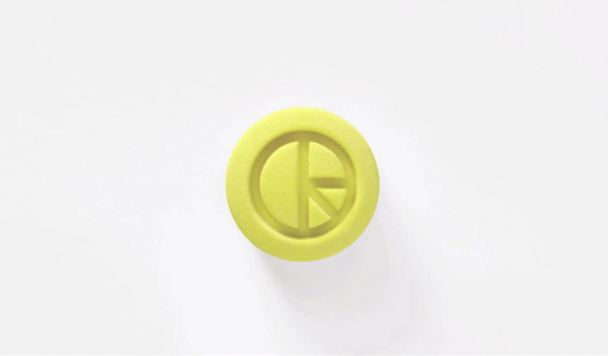The image showcases a detailed photograph of a yellow, circular, cylindrical object set against a seamless, white background. Viewed from a bird's eye perspective, the object appears three-dimensional and textured, possibly made of plastic or rubber, and resembles a button or a key component with an indeterminate function. The intricately designed logo or symbol is prominently featured in the center, carved into the object. The outer edge forms a circular indent, within which lies a series of distinctive carvings: a line bisects the circle vertically, and additional lines create sectional divisions akin to pie slices on the right side. These divisions result in one semicircle on the left, one quarter-circle on the top right, and two eighth-circle sections on the bottom right, collectively resembling a lowercase "k" intersecting a circle. A slight shadow casts to the bottom right, hinting that the lighting originates from the top left off-screen, enhancing the object's depth and texture.